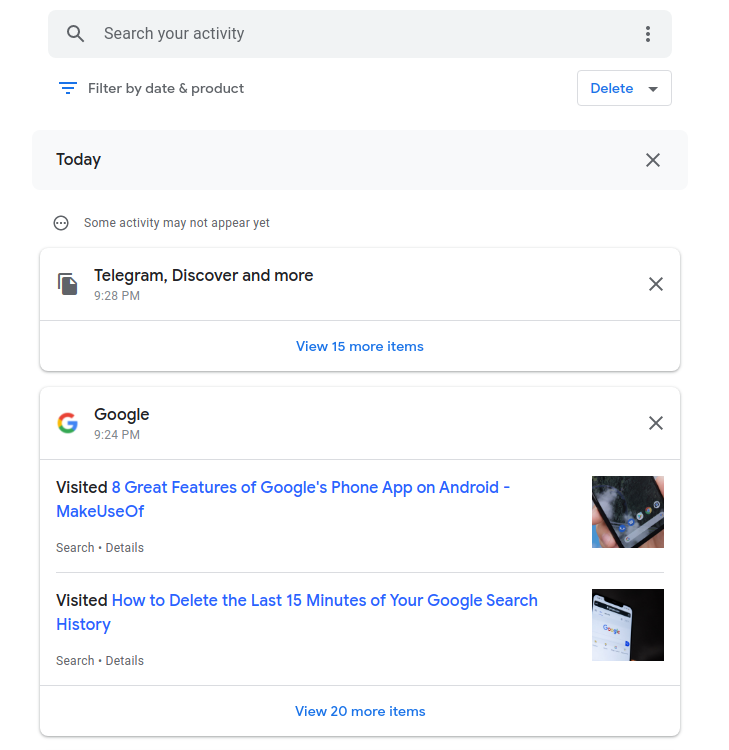The image is a screenshot from a desktop displaying the "My Activity" page in Google settings. At the top, there's a search bar with the placeholder text "Search your activity" and a magnifying glass icon. To the right, there are three vertical dots indicating additional settings, and below these dots is a delete option.

Underneath the search bar, there's a filter option labeled "Filter by date and product." The display shows activity from today, specifically detailing Telegram and Discover interactions at 9:28 PM. A note beneath this indicates that some activity may not appear yet, with a prompt stating "15 more items" that can be viewed if desired. There's also an option to close the note with an 'X' in the top right corner.

Further down, the screenshot reveals specific activities: 
1. A visit to an article titled "8 Great Features of Google's Phone App on Android" from "Make Use Of."
2. A visit to a tutorial on "How to Delete the Last 15 Minutes of Your Google Search History."

There is another option to view "20 more items." The image suggests a user's recent search activities possibly involving concerns about search history privacy.